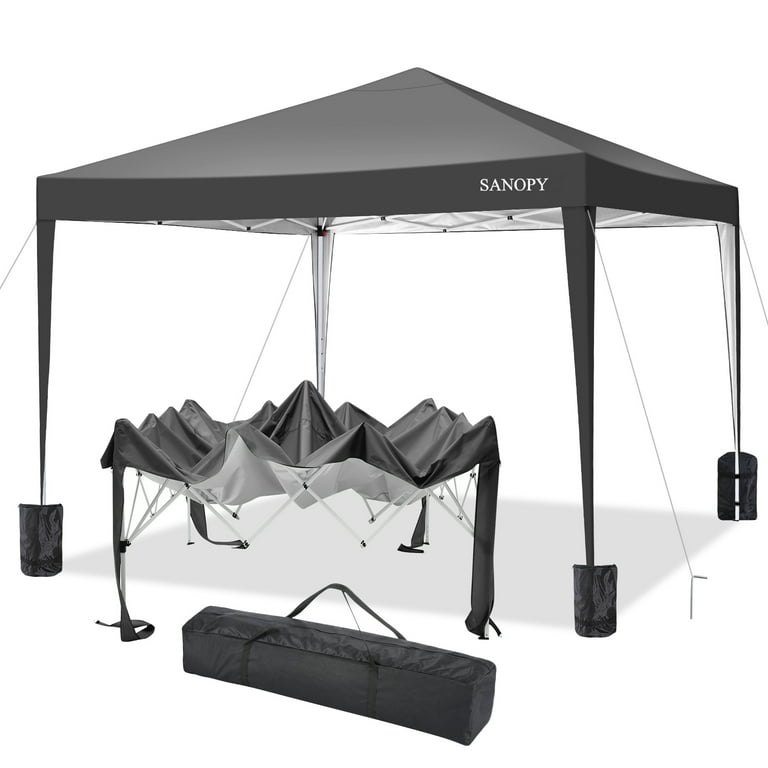The image depicts a marketing-style photograph of a large, wall-less canopy or party tent, suitable for festivals or street fairs. The photograph is isolated on a pure white background and is presented from a three-quarter angle, showing the canopy facing left. The tent has a dark green or black peaked triangular roof supported by four tall metal poles. Each pole is encased in a weight or pot at the base, securing the canopy to the ground. The canopy bears the brand name "SANOPY" in white, capital letters on the right corner of the roof. 

The main image is complemented by two smaller images below it. The first smaller image shows the same canopy in a semi-folded state, giving a visual representation of what it looks like before being fully erected. The final image at the bottom illustrates the canopy completely packed into a small, rectangular carrying case with two handles, highlighting its portability. The organized sequence of these images effectively demonstrates the canopy's setup, partial closure, and compact storage.